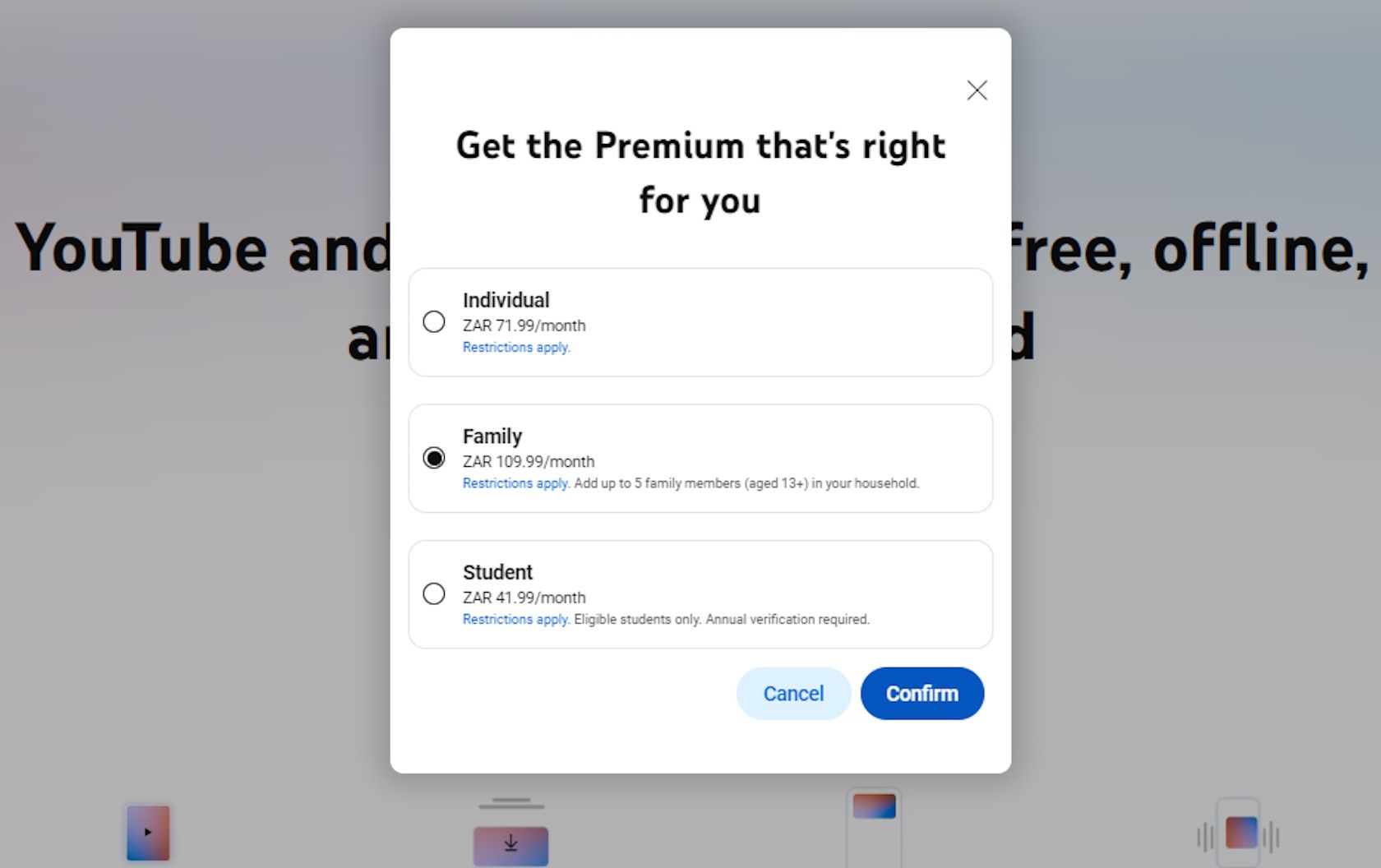In the center of the image, a prominent pop-up menu dominates, obscuring the underlying main page. The pop-up menu features a clean, white background with primarily black text, except for the emphasized words "Restrictions Apply," which are likely highlighted for attention.

At the top of the menu, a heading reads, "Get the premium that is right for you," inviting users to select from three premium options. Each option includes a checkbox for selection:
1. **Individual**: Priced at 71.99 ZAR per month, this option notes that "restrictions may apply."
2. **Family**: This plan costs 109.99 ZAR per month and allows the addition of up to five family members as part of the household, with an emphasis that "restrictions may apply." This option is currently highlighted, indicating it is selected.
3. **Student**: Available for 41.99 ZAR per month, this plan is exclusive to students and requires annual verification. Again, "restrictions may apply."

At the bottom right of the pop-up menu, there are two blue buttons labeled "Cancel" and "Confirm," providing navigation choices for the user.

In the background, partially visible behind the pop-up, the main page exhibits some text, with "YouTube" and the phrase "Free Offline" perceptible, hinting that the subscription service being offered is related to YouTube.